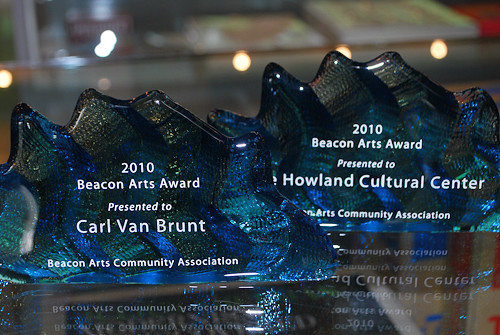Two transparent, bluish-green acrylic awards sit on a shiny, reflective glass surface. The awards have a unique design, resembling a blue shell with three ridges in the center and an element rising on the far right side. The left award reads "2010 Bitcoin Arts Award presented to Calvin Brunch" and at the bottom, "Bitcoin Arts Community Association" in white font. The right award similarly states "2010 Bitcoin Arts Award presented to Howland Cultural Center," with "Arts Community Association" partially visible at the bottom due to the left award's positioning blocking part of the text.